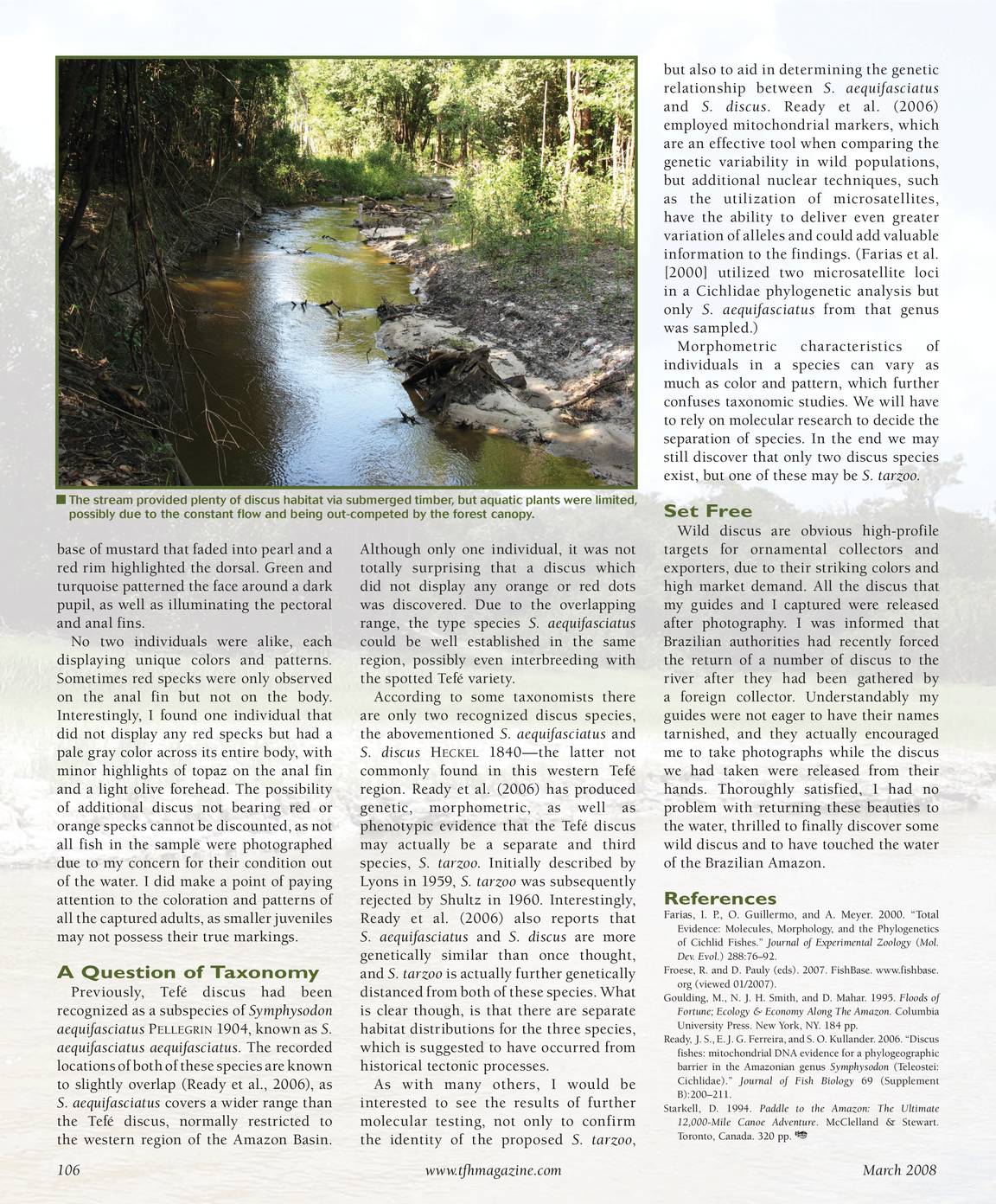This image is a detailed scan of page 106 from the March 2008 issue of TFH Magazine with the website www.tfhmagazine.com at the bottom center. The page is filled with black text arranged in three columns, and it features an upper-left photograph of a stream surrounded by various plants. The accompanying caption reads, "The stream provided plenty of discus habitat via submerged timber, but aquatic plants were limited, possibly due to the constant flow and being out-competed by the forest canopy." The stream appears greenish, with light shining off its surface, bordered by dirt, rocky banks, and green shrubs, while bare tree limbs and sticks jut out of the water. The photograph is framed by additional details, including references in the lower right and a few paragraph headings, such as "A Question of Taxonomy" and "Set Free." This comprehensive article seems to explore the discussion surrounding a subspecies identified in 1904, known as telodiscus.